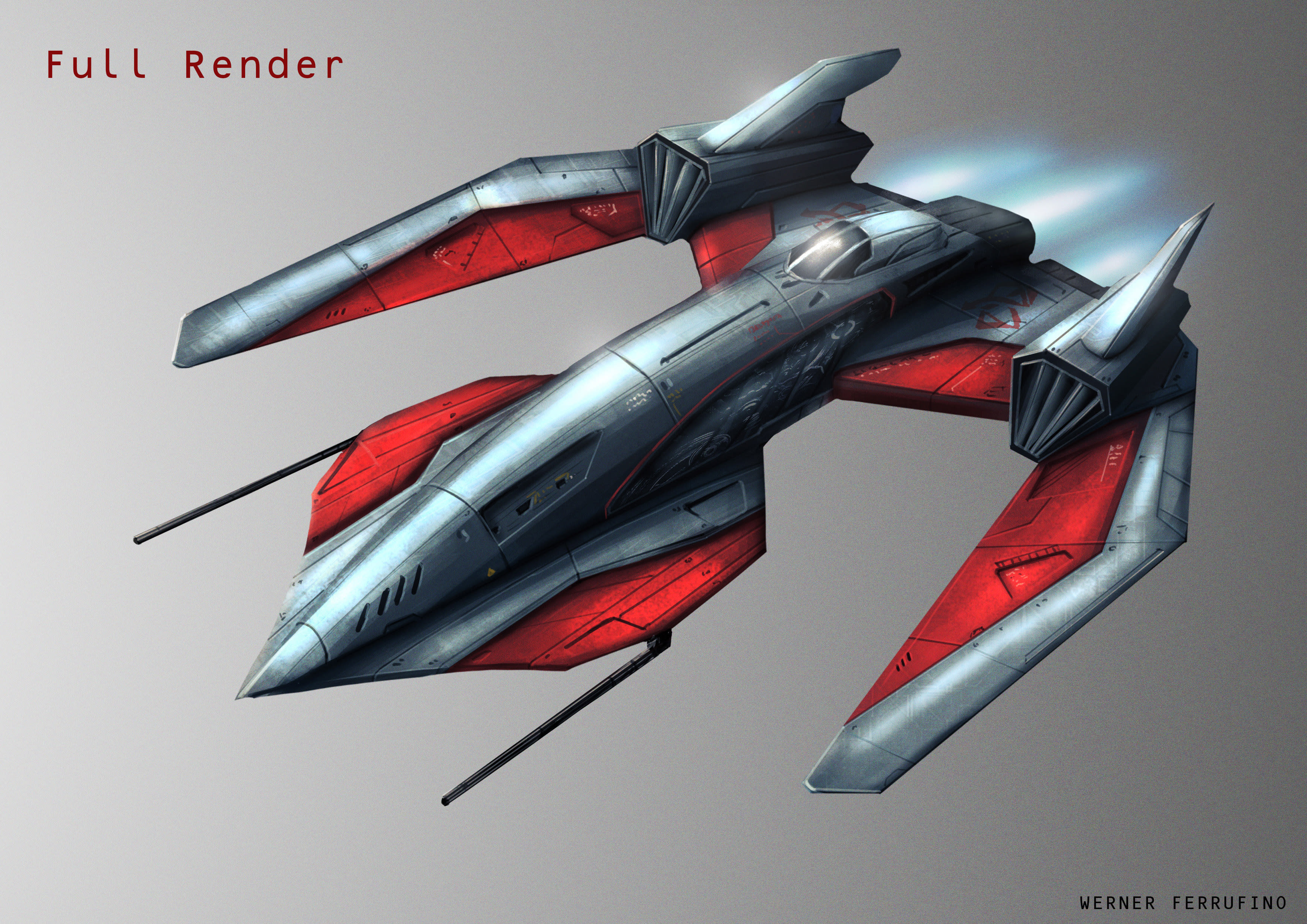This detailed digital render depicts a futuristic spaceship, likely designed for a science fiction video game or movie. The spaceship has a distinctive U-shaped, or W-like, design with three prongs; the outer prongs extend downwards and are equipped with motors and small fins at their ends. Its body is a sleek metallic silver, accented with vivid red sections. Detailed blackened windows form the cockpit towards the rear middle, leading up to the pointed nose of the craft. Additionally, two long, slender black stick-like appendages, resembling guns or lasers, extend from the front. A bright blue flame thrusts from the back, indicating motion. The image features a gray background with "full render" written in red in the upper left corner, and "Werner Ferufino" written in black in the bottom right corner.